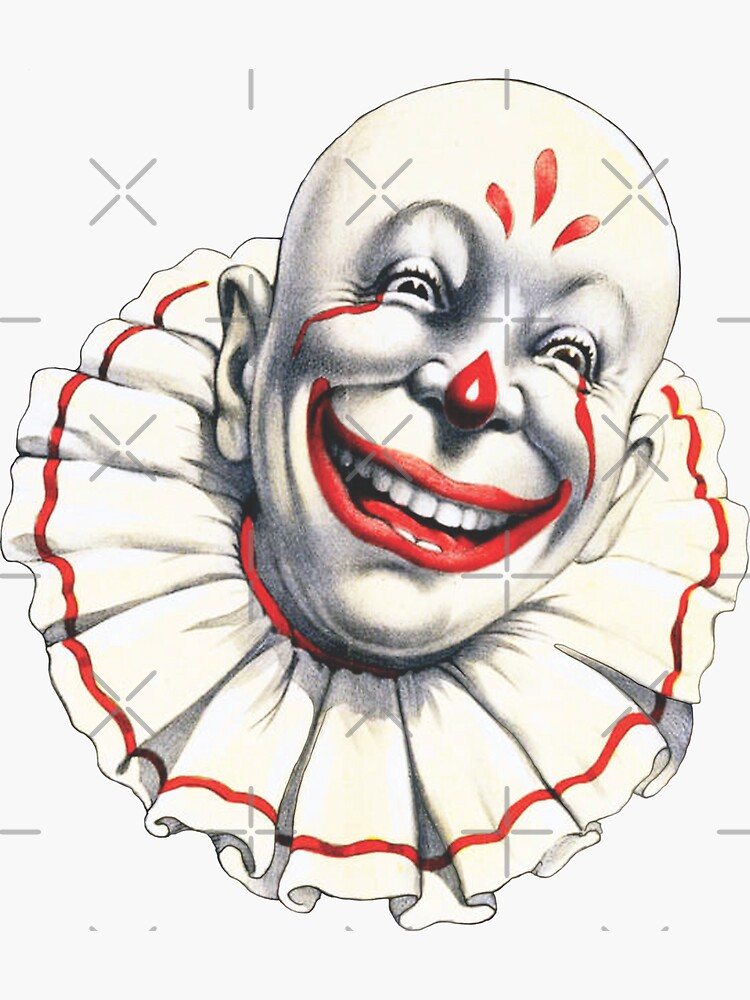This is a drawing of a happy animated clown on a white background, distinguished by a light gray watermark running across it. The bald clown features three red, teardrop-like shapes on its forehead, and from its eyes, red lines resembling tears run down. Its nose has a red drop, typical of clown imagery, though not fully covering the nose. The clown has a very wide red mouth that exposes white teeth and a hint of a tongue underneath. Its ears are light gray in color. Surrounding the clown's neck is a frilly, circular white scarf trimmed with a thin red border. The clown appears primarily in black, white, and red, and the overall expression of the clown is joyful, with little black eyelashes enhancing its animated and cheerful demeanor.